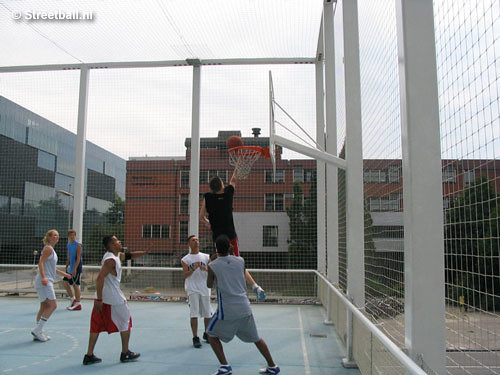This photograph captures a lively street basketball game played on an outdoor court nestled within an urban setting. The court, featuring a light blue floor marked with white lines, is enclosed by a chain-link fence supported by white metal posts, providing a secure play area. High mesh netting, also held up by white pillars, surrounds the court to prevent the ball from escaping. The image includes four men and one woman, all dressed in typical basketball attire consisting of sleeveless t-shirts and long shorts in shades of white, gray, blue, and black, along with tennis shoes. The player wearing a black shirt is seen mid-air, executing a layup towards the hoop positioned at the center of the photo. The background reveals elements of the urban environment, with a parking lot, a glass-faced building, and a red brick building, possibly modern apartment blocks or a school, rising about four stories high. In the upper left-hand corner, the photo is annotated with the copyright "streetball.nl," indicating the scene is likely set in the Netherlands.